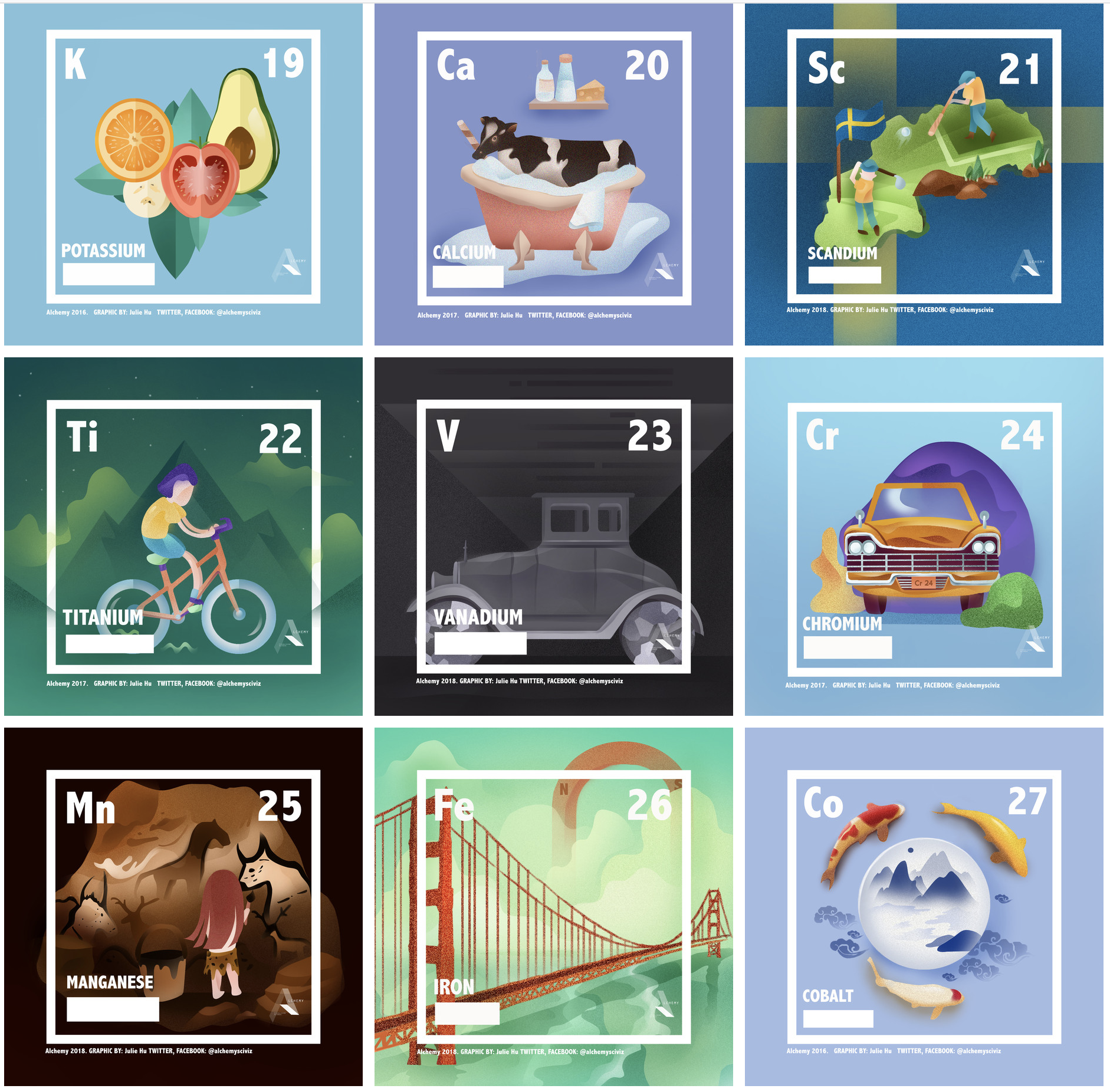The image is a detailed computer graphic of nine elements from the periodic table, arranged in a 3x3 grid. Each square features the standard element notation with additional illustrative backgrounds related to the respective elements. The top left square represents potassium (K-19) in a blue frame featuring fruits like an orange, tomato, and avocado. The top middle square is for calcium (CA-20) in a purple frame showing a cow in a bathtub. Scandium (SC-21) occupies the top right with men playing golf and a Swedish flag in the background. 

In the middle row, the left square is for titanium (TI-22) marked by a person riding a bicycle. The center square represents vanadium (V-23), depicted with a vintage black-and-white car. The right square is chromium (CR-24), featuring an orange car driving towards the viewer. 

The bottom row includes manganese (MN-25) on the left, showing an indistinct image resembling cave drawings. In the middle, iron (FE-26) is highlighted with the iconic Golden Gate Bridge in the background. Finally, cobalt (CO-27) in the bottom right square is illustrated with three fish swimming around a circle with mountains in the backdrop.